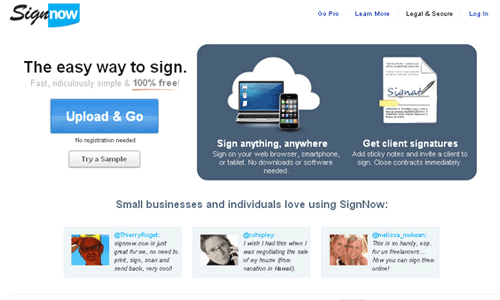In the image from the post, a prominent advertisement for the application "SignNow" is displayed. The SignNow logo is distinctive, with 'Sign' written in black and 'Now' in white lettering against a blue background, making it stand out. The advertisement headline touts "The easy way to sign," written in black ink, while below it, in faded grey ink, the benefits are listed as "fast, ridiculously simple, 100% free, upload and go." The ad suggests downloading the application onto your computer or phone, though it cautions about having virus protection. 

A dark blue-grey box contains more promotional material. Inside, there are images of a smartphone and laptop, emphasizing that users can "sign anything, anywhere," using their web browser, smartphone, or tablet without needing downloads or software. Adjacent to these images, there is a PNG of a document, likely a legal one, being signed. Below, it states users can "get client-held signatures, add sticky notes, and invite clients to sign," thus facilitating the immediate closing of contracts. This service seems tailored to professionals involved in legal, business, or notary work who require secure and efficient electronic signature solutions.